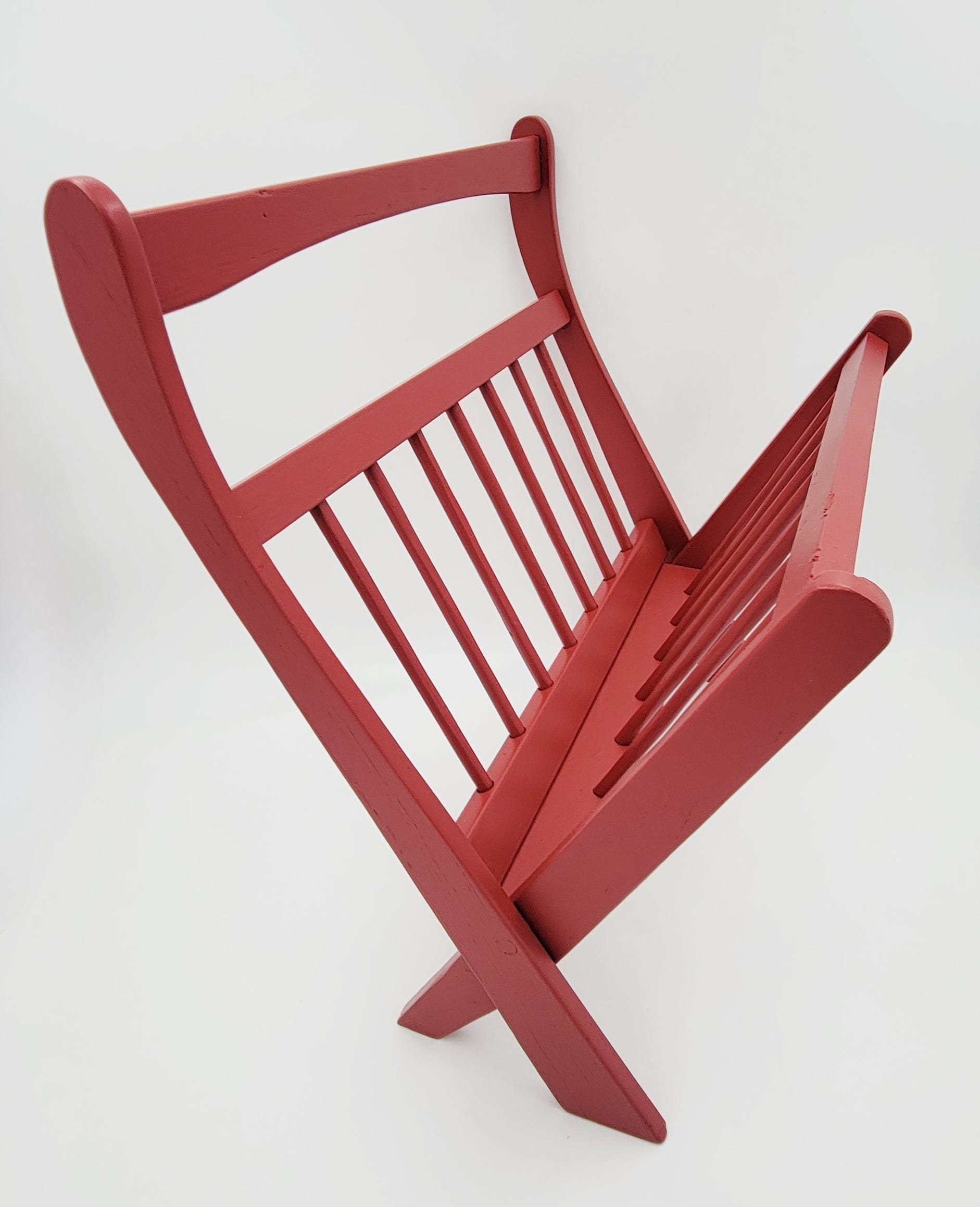The image features a vintage red wooden newspaper rack, likely hand-painted. The design is reminiscent of old-fashioned styles not typically seen in modern homes. The rack consists of eight spindled bars on each side and is hinged in the middle, allowing it to fold flat for storage or open up into a V-shaped stand with crisscross legs. The red paint is chipped in places, suggesting frequent use over time. The photograph is set against a stark white background, providing no contextual clues whether it's placed in a home or displayed for sale. It's empty and meticulously centered, highlighting the stand's functional and aesthetic characteristics.